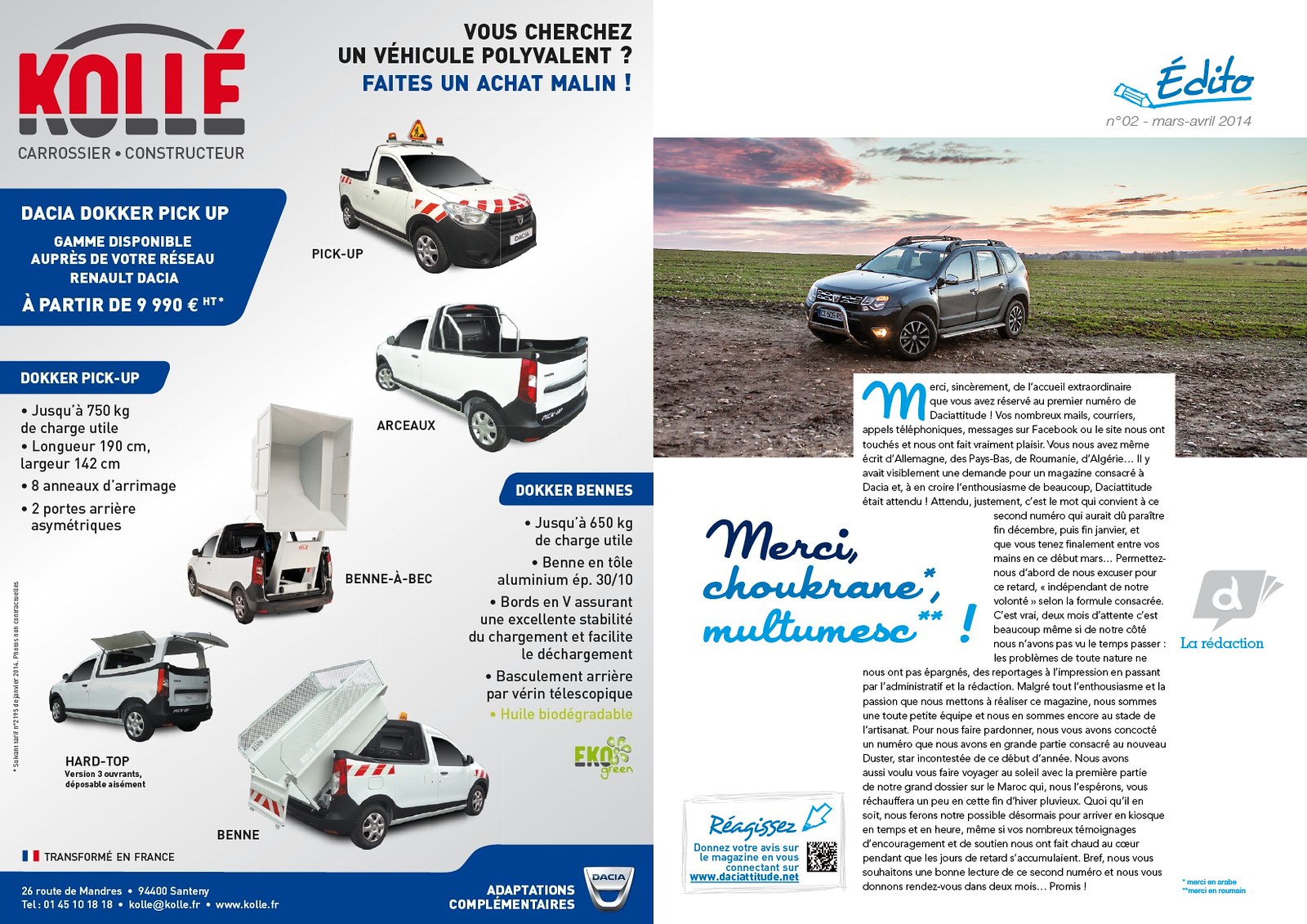The image is a detailed French brochure for the car brand KOLLE, prominently featuring their versatile truck models and an SUV. On the left side of the brochure, there are multiple images showcasing five different configurations of the KOLLE truck: a basic pickup, the Arso, Benet aback, Hardtop, and another Benet variant, each displaying diverse functionalities such as having an open bed, a dump truck conversion, and a hardtop cover. Accompanying these images are bullet-point lists of specifications and features in French, under blue headers, with a red and gray KOLLE logo in the upper left corner and additional black and blue text in the upper right corner. The bottom left of the panel shows a small French flag and contact information formatted as an address and telephone details. 

On the right side of the brochure, there is a picture of a sleek gray SUV parked on a grassy, gravelly road against a backdrop of a stunning sunset sky. This page also includes a lengthy article in French, written in black text with emphasized quotes in flowing, cursive blue text. The layout is detailed, with a blue border at the bottom containing white text, all aimed at providing comprehensive information for potential buyers.